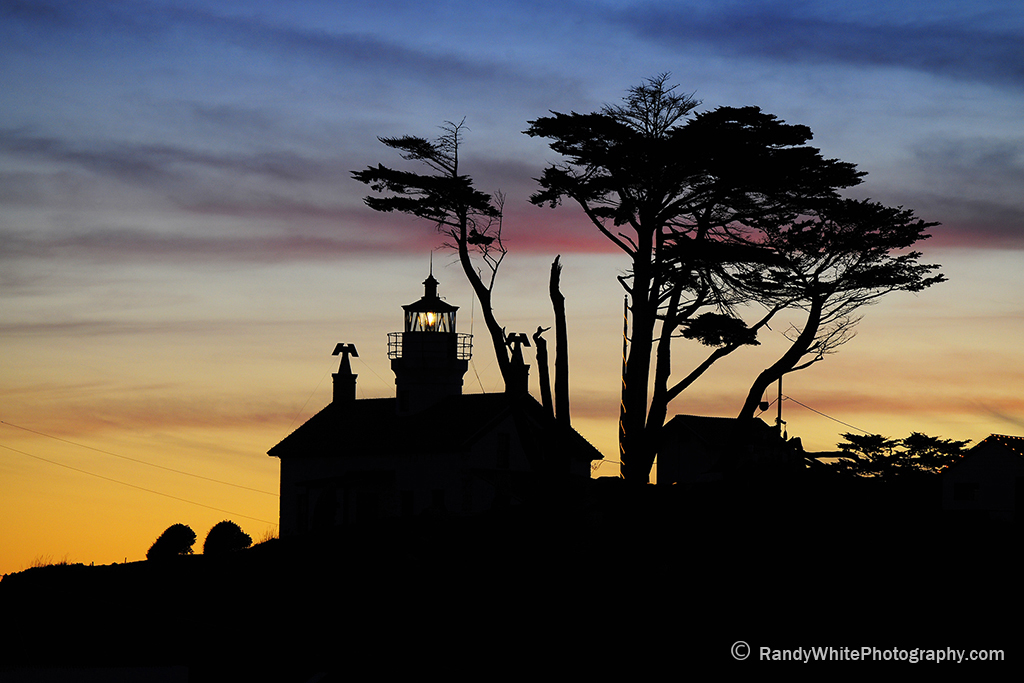Against a mesmerizing backdrop of a vibrant night sky, this captivating photograph by Randy White captures a richly detailed silhouette scene. The sky transitions through an array of stunning colors: streaks of blue and violet dominate the top, shifting into red and purple hues, with pale lilac and peach bands gradually blending into yellow near the horizon. 

In the foreground, a low-lying house emerges in stark silhouette. Its defining feature is a miniature lighthouse positioned on the roof, complete with an encased wire balcony and a luminous center. To either side of the rooftop, mounted on pillars, are sculptural elements that resemble bird wings. 

Adjacent to the house stands a prominent deciduous tree with a complex structure of multi-trunk branches, some ending in vibrant green leaves while others remain bare. Smaller trees and bushes pepper the scene, enhancing the intricate silhouette against the sky's luminous gradient. The ground below is pitch black, emphasizing the dramatic contrast of the silhouettes. At the bottom right corner, the photograph is credited to RandyWhitePhotography.com.